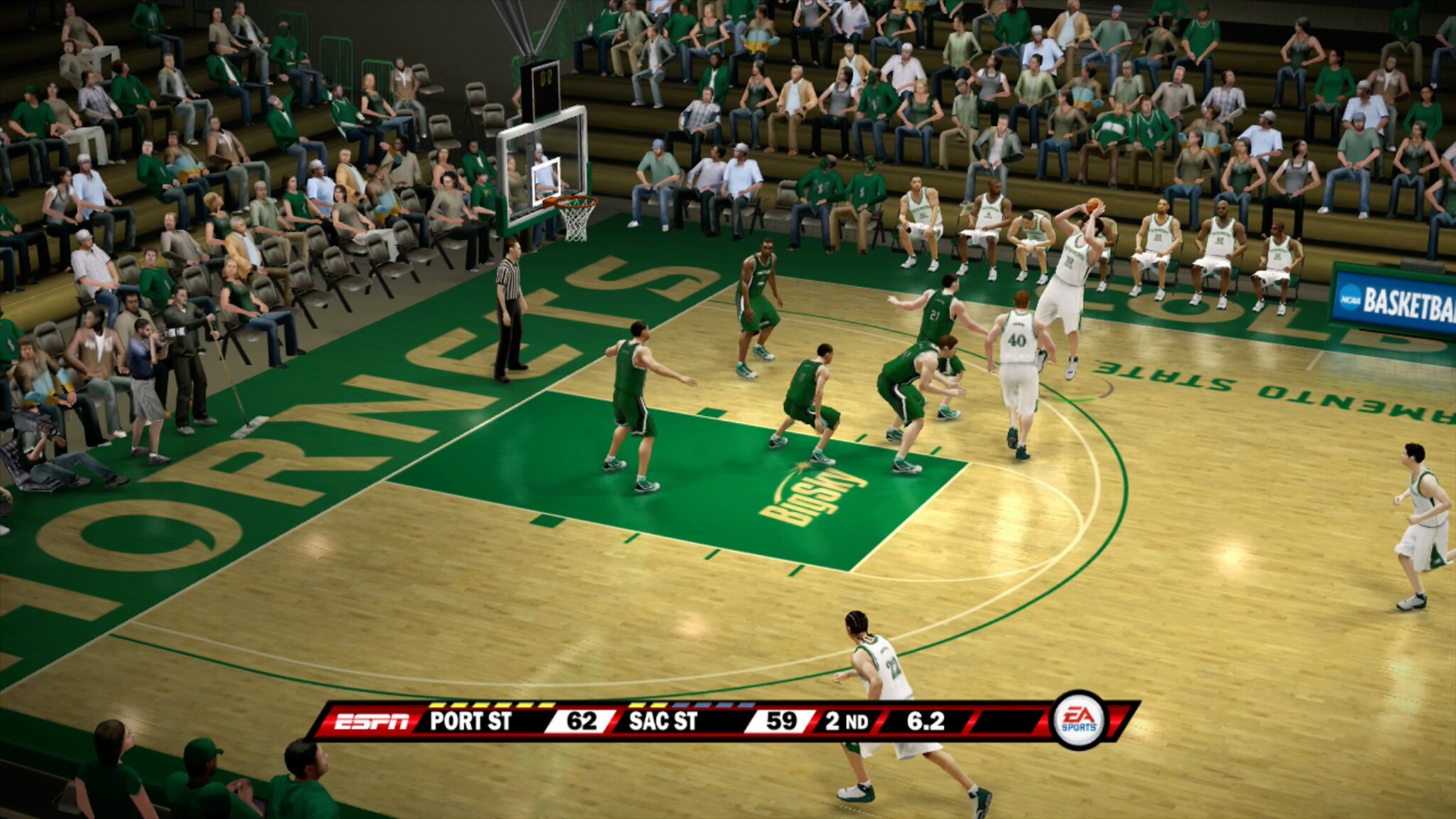This meticulously crafted computer-generated image captures the dynamic essence of a basketball game set within an expansive gymnasium or arena. The light wooden floor glistens under the radiant overhead lights, casting subtle reflections that enhance the sense of liveliness on the court. To the left, players sport vibrant green shorts and tops, while their opponents on the right are clad in crisp white uniforms. 

The audience forms a vibrant backdrop, with spectators seated both straight ahead and along the left-hand side, their expressions and movements hinting at the excitement of the game. In the foreground, three individuals are seated on chairs in the lower left corner, their attention focused intently on the action unfolding before them.

A referee, positioned towards the left-hand center of the court, ensures the game adheres to the rules as the players engage in the fast-paced athletic competition. The basketball net on the left side stands as the target for the players' intense efforts. A scoreboard at the bottom of the image keeps track of the progress, further immersing viewers in the thrilling atmosphere of this simulated sporting event.